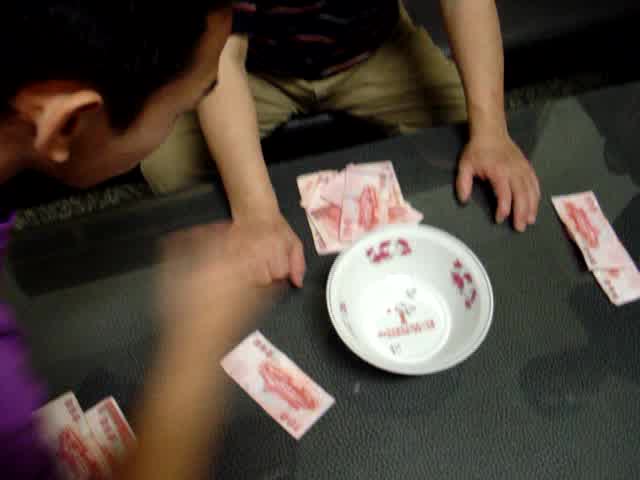A somewhat blurry image captures two individuals engaged in a scene. The person on the left, appearing to be of Asian descent with brown skin, is shown in profile. Their distinctive large right ear and a glimpse of their purple shirt are visible, along with their right hand, which seems blurred and is held up to the middle of the frame. On the right, a second individual with white skin is seated, facing the camera. Only the bottom half of their torso, their legs, and hands are visible. They are manspreading, wearing an olive green pants and a black shirt. Their hands rest on a greenish-gray table. Central to the image is a white bowl adorned with red designs and an indiscernible red text or image at its center. Scattered on the table are several white currency bills, each featuring red text and images. Two bills are positioned to the right of the person's left arm, four between their arms, one bill near the bottom of their right arm, and two overlapping bills sit in the bottom left corner near the individual in the purple shirt.